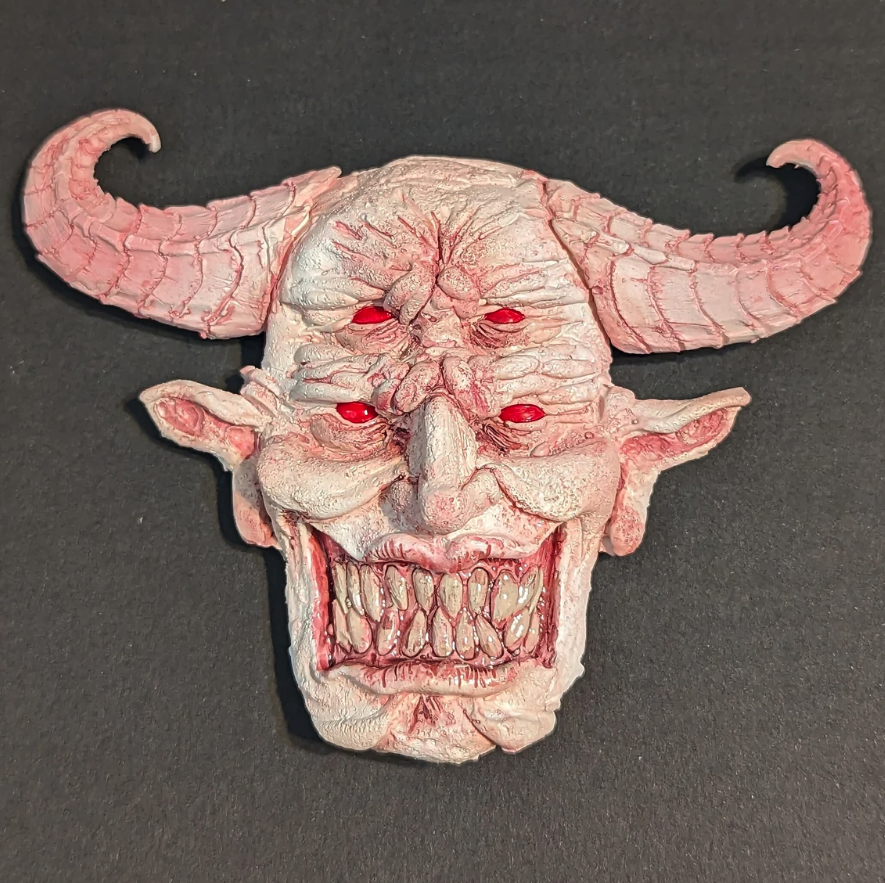The image showcases a detailed, eerie demon mask positioned prominently in the center of the frame. The mask is composed of a mixture of red, pink, and white hues, which blend seamlessly to create a haunting, otherworldly vibe. It features two curled horns on top of the head, adding to its menacing appearance. The demon's face is striking with four gleaming eyes; two are situated on the forehead, while the other two are in the expected eye sockets. Below the eyes is a defined nose, flanked by elongated, elf-like ears. The mask's mouth is wide open, revealing jagged, off-white teeth set against pink gums, giving it a menacing grin. The object is laid out on a dark, possibly tiled background, which enhances the unsettling contrast of its colors. The background's off-white and charcoal black or gray tones further emphasize the vivid details of the mask's demonic features.